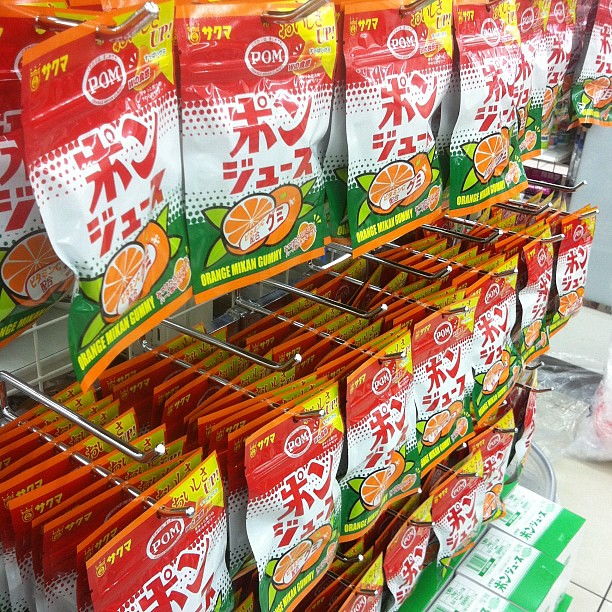This detailed image was taken in a retail or convenience store, likely an Asian grocery store. It features a wall display of orange gummy candies packaged in distinctive red, white, and green bags. The bags prominently feature pictures of oranges and the text "orange milk and gummy" in yellow. Central to the design is a white band with Chinese characters in red. The branding at the top reads "POM." The packaging also includes holes at the top, which allow the bags to hang from hooks on a grid rack. There are multiple rows and columns of these candies, organized neatly across approximately seven rods, creating an appealing and colorful display of Asian snacks.